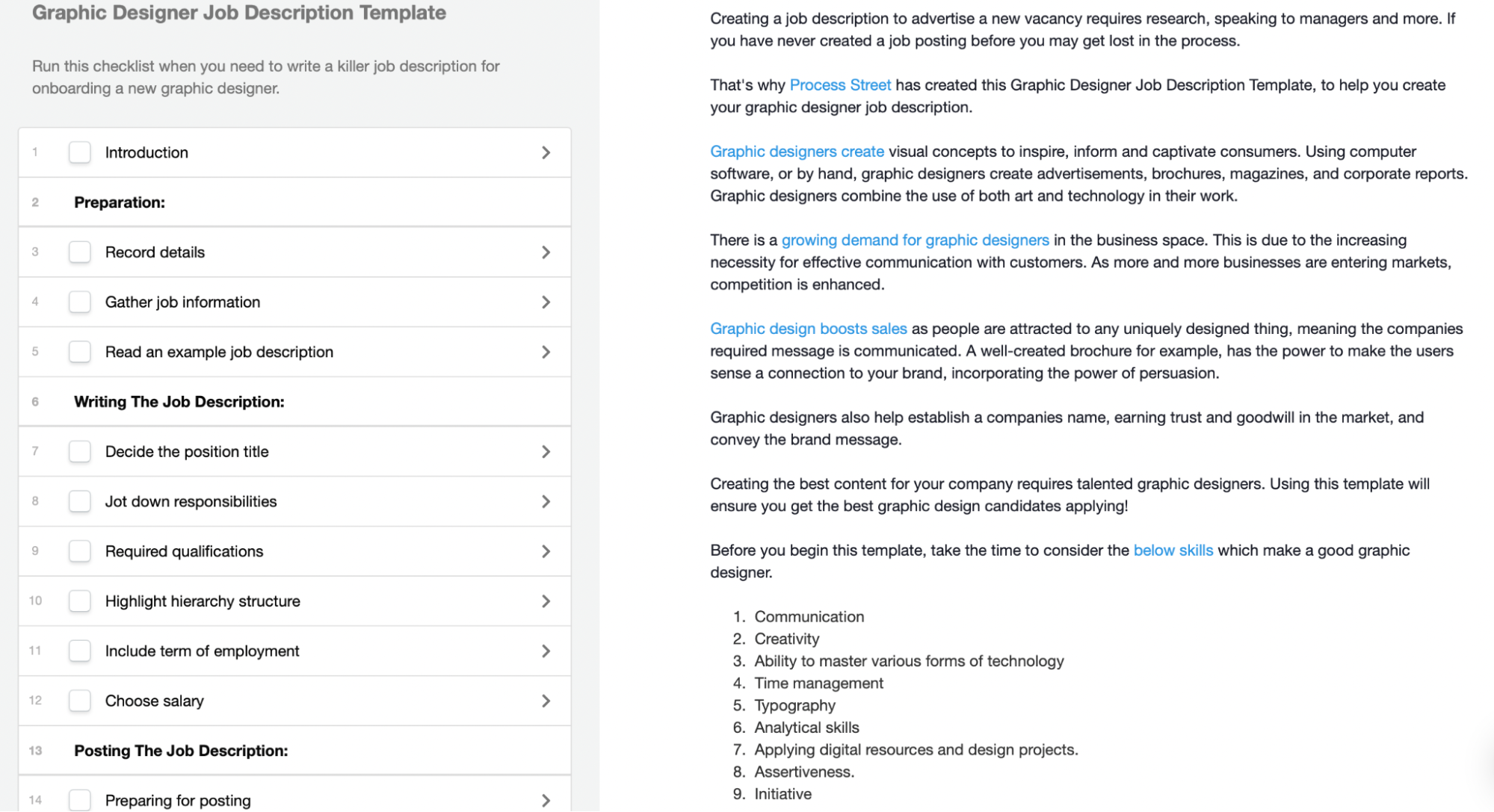This image is a detailed screenshot of a dashboard interface designed for editing a page, specifically tailored to creating a Graphic Designer Job Description Template. The left side of the interface features a gray vertical panel. At the top of this panel, prominent text reads "Graphic Designer Job Description Template." Directly beneath this heading is an informative subtitle, indicating: "Run this checklist when you need to write a killer job description for onboarding a new graphic designer."

Below this explanatory note, a structured list of actionable buttons is neatly arranged. Each item in the list is accompanied by a checkbox on the left side, suggesting tasks need to be completed sequentially. To the right of each task, a forward arrow icon is present, likely indicating further sub-tasks or additional information.

The tasks listed in the checklist are as follows:
1. **Introduction**
2. **Preparation**
3. **Record Details**
4. **Gather Job Information**
5. **Write an Example Job Description**
6. **Writing the Job Description**

This well-organized dashboard provides a comprehensive guide through each step necessary for crafting an effective job description for a new graphic designer, ensuring all critical elements are covered systematically.